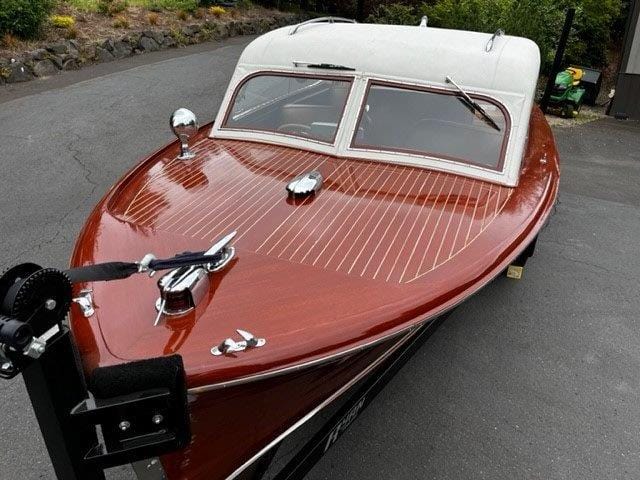This image showcases a vintage-styled speedboat, prominently featuring a glossy burgundy-red body adorned with fine white lines. The boat's front section, enhanced by a chrome hood ornament and anchored with a black device likely used for towing, sits on a gray asphalt driveway. The overhead area, intended for the captain and passengers, is covered by a white canopy, featuring two windows with visible seats inside. Distinctive chrome elements, including windshield wipers on the white windshield and mirrors, add to its retro charm. Surrounding the boat, the background reveals patches of grass, stones, shrubs, and a few trees, as well as a green machine on the right side, contributing to the outdoor setting.